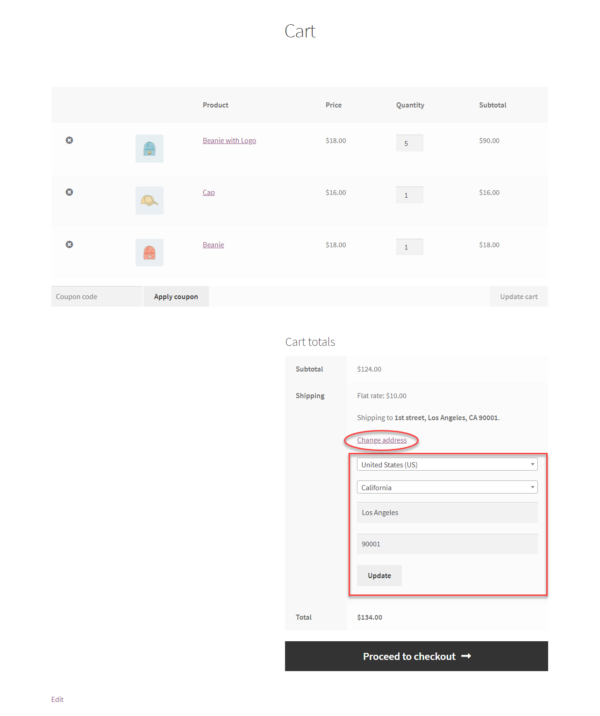A detailed image shows a shopping cart interface with a white background. The cart section lists three items, each with detailed information including the product name, price, quantity, and subtotal. Below this, a smaller block displays the cart totals: a subtotal of $124, a flat shipping rate of $10, and the designated shipping address to 1st Street, Los Angeles, CA 90001, highlighted in red. There is an option to change the address. Underneath, a red box displays the country, state, city, and zip code for shipping, all listed as United States, California, with options to change these details. A button below labeled "Update" adjusts the shipping details if needed. The total amount, including shipping, sums up to $134, followed by a "Proceed to Checkout" button.